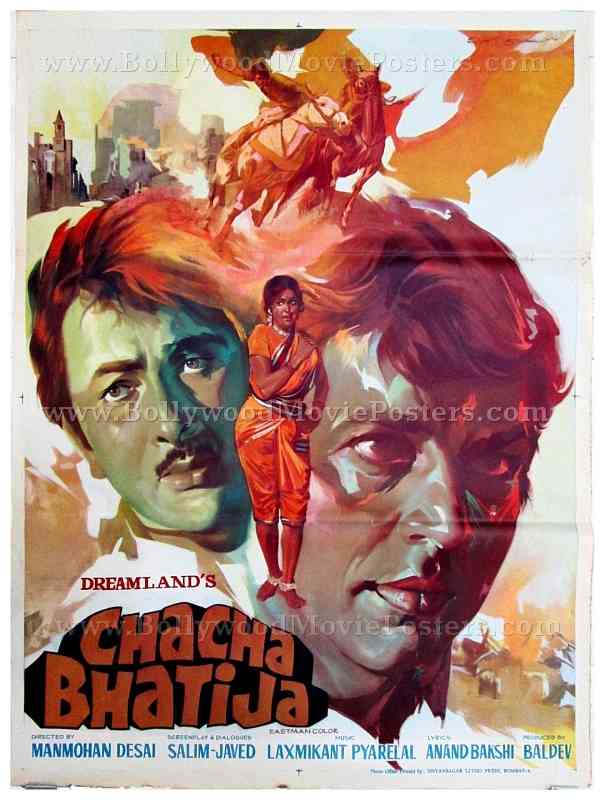This vibrant and eye-catching poster for the Bollywood movie titled "Chacha Bhatija" from Dreamlands depicts intricate and lively artistry, reminiscent of impressionist or watercolor styles. The website www.BollywoodMoviePosters.com is prominently displayed as a watermark across the center. The bottom portion of the poster lists the actors' names in blue capital letters, enhancing the colorful theme with hues of oranges, reds, purples, blues, greens, and yellows.

The central figure of the poster is an Indian woman dressed in an orange sari, standing gracefully between the large illustrated faces of two men. One man's portrait, more dominant, looks to the right, while the other man is slightly smaller and glances to the left. Above these figures, two horses, one white and one brown, appear to be galloping, adding dynamic movement to the scene. In the background, a cityscape emerges, contributing to the poster's depth.

This poster's artistic rendition, complete with visible brushstrokes and fold marks, gives it a nostalgic yet engaging appeal, ensuring it would capture attention if seen on a wall. The combination of detailed imagery and vibrant colors encapsulates the essence of Bollywood's cinematic vibrancy.